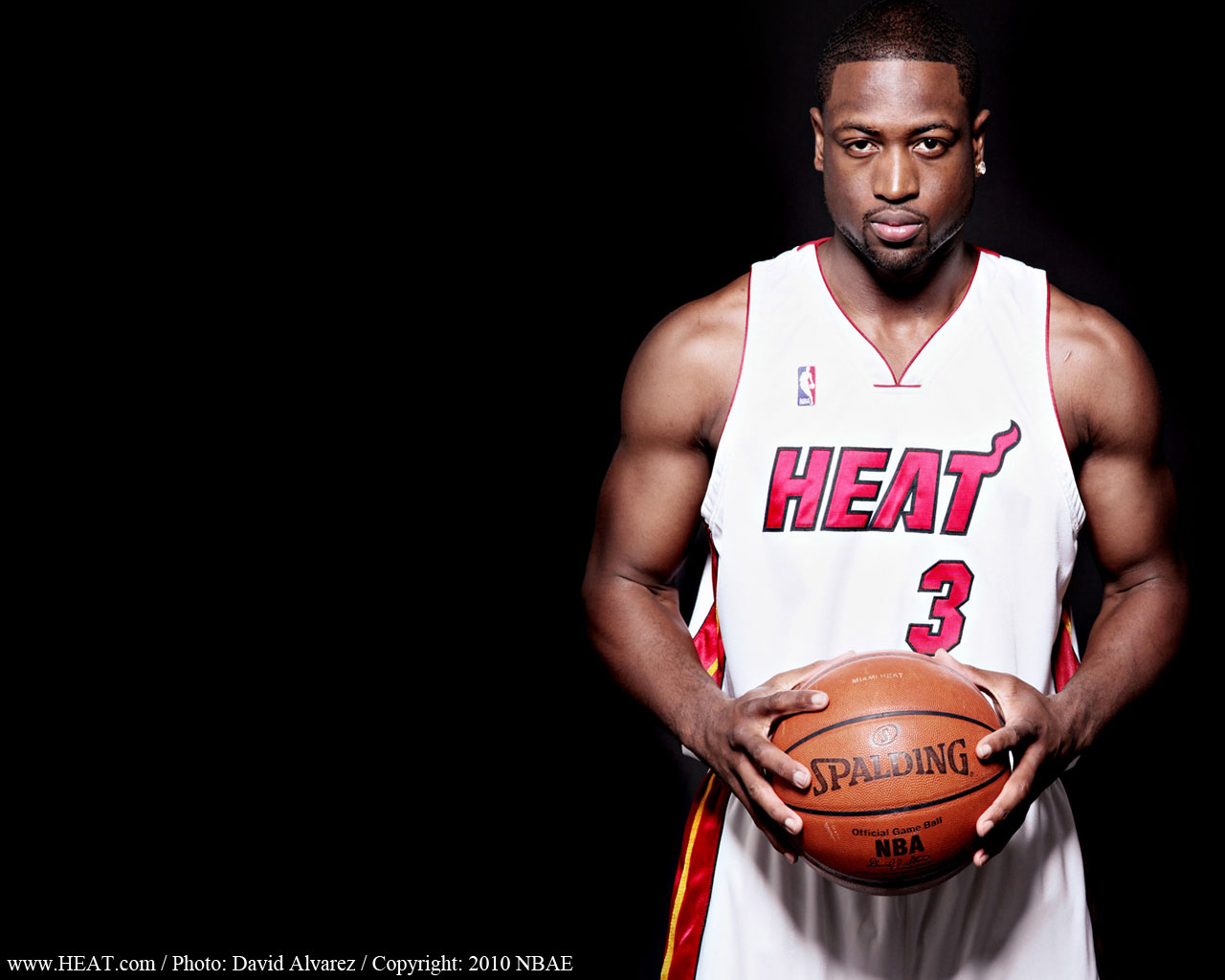Set against a jet black background, this image features a basketball player prominently on the right side. The player, an African American man, is standing facing forward, holding a basketball with both hands in front of him. The ball, labeled with "Spalding" in black and "NBA" below it, is centered in the image. He sports very short black hair, a faint mustache, and a thin goatee, along with a large diamond earring in his left ear. 

He is clad in a distinctive Miami Heat jersey, white with the word "Heat" in reddish letters across the chest and the number three in red below it. The NBA logo is visible on the right side of the chest. His shorts, predominantly white, feature yellow and red stripes down the side, though they are cut off just above the knees in the photo. 

In the bottom left corner of the image, there is white print that reads "www.heat.com.photo.DavidAlvarez.copyright2010NBAe." Given the details, the player in the photo appears to be Dwyane Wade.